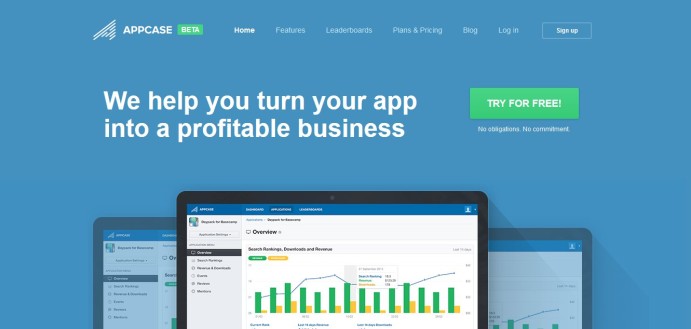The image is a horizontal screenshot of a webpage, focusing on the top portion. The background is a medium sky blue color. In the upper left quadrant, the brand's name "AppCase" is displayed alongside an icon. To the right of the brand name, there is a button labeled "Beta." 

The navigation menu features small white text headings that include "Home," "Features," "Leaderboards," "Plans and Pricing," "Blog," and "Login." Additionally, there is a "Sign Up" button. The "Home" section is selected, indicating this as the homepage. 

The main content area displays a large white font headline stating, "We help you turn your app into a profitable business." Below this headline, there is a green "Try for Free" button. Underneath the button, in very small text, it reads, "No Obligations, No Commitment."

The central visual element is the top part of a laptop screen, showing two charts. The laptop screen is partially obscured on the left and right by shadows of other screens, creating a sense of depth. The main screen in the center displays charts in green and yellow with a blue header bar and white dropdown buttons at the top of each chart.